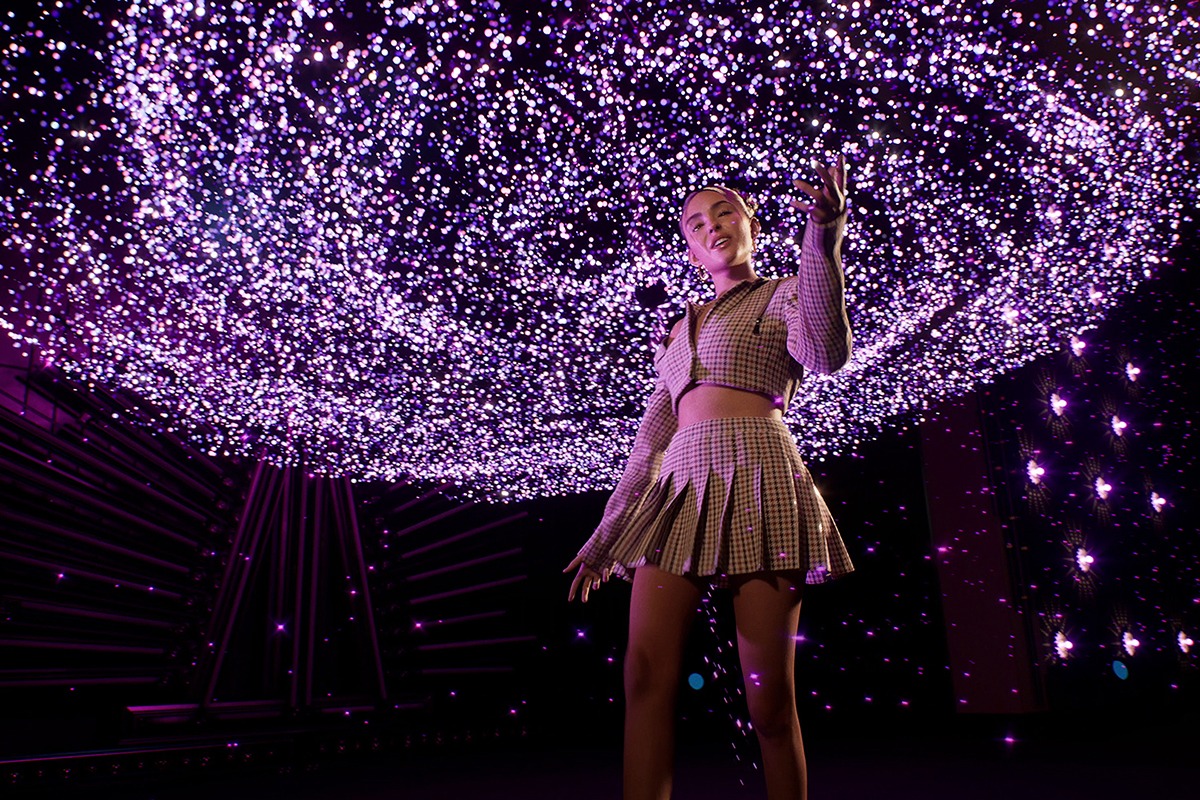In this striking photographic image, a young white woman in her 20s commands the frame from an indoor setting, lit with a captivating violet hue. She stands with her hips slightly twisted, legs apart, wearing a fashionably cropped jacket with long sleeves that reveals her midriff. The outfit is completed with a short skirt that flares approximately 18 inches above her knee. Her hair is pulled back, with a few loose strands framing her face.

Her pose is dynamic: her left hand rests by her skirt while her right arm is raised with fingers outstretched. She gazes downward at the camera from a high vantage point, suggesting the photograph was taken from below, possibly from a kneeling position.

Behind her, an almost surreal background evokes a cosmic landscape, resembling a Milky Way galaxy with a swirl of stars stretching from the top left to the center of the image. These stars form a captivating pattern, like a celestial tornado. On the right side of the background, a series of vertical and horizontal marks, reminiscent of partially completed plus signs, adds a unique geometric texture. The entire scene is bathed in a purple glow, enhancing the ethereal quality of the visual.